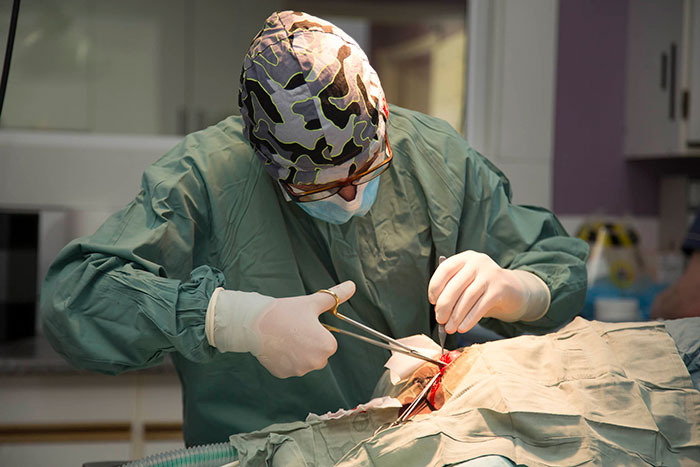This image captures a detailed and intense surgical operation being performed by a surgeon in an operating room. The central focus is on the surgeon, who is dressed in green scrubs and wearing white latex gloves, engaged deeply in the procedure. His head is adorned with a camouflage cap, and he is also equipped with black glasses and a surgical mask that covers his face. The surgeon is intently looking down at the incision, which is clearly visible on the patient's body beneath a surgical drape, with some red seeping through the cloth indicating the site of surgery. In his hands, the surgeon holds a pair of scissors in his right hand and a pair of tweezers in his left, precisely working at the incision. The patient lies on the operating table covered with blue surgical cloth. Behind the surgeon, a purple-painted wall is visible along with a window featuring a white frame, and adjacent white cabinets contribute to the sterile, clinical atmosphere of the room.